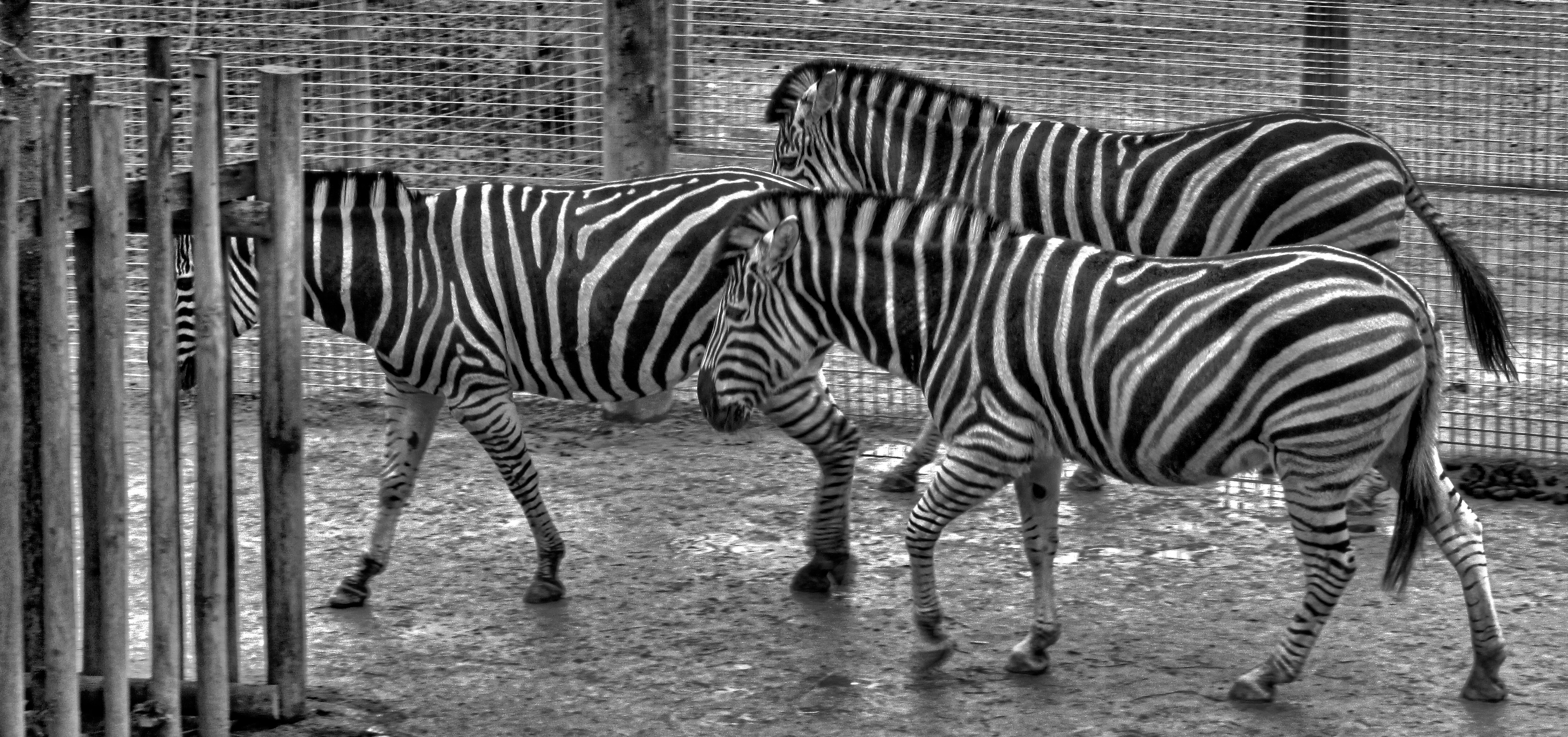This detailed black and white photograph captures three zebras walking from right to left. The zebras are in motion, with the two on the right side mirroring each other's steps, while the one on the left is slightly ahead. To the left, a wooden fence extends horizontally, partially obscuring the head of the foremost zebra. The ground they tread on is muddy, featuring visible puddles that suggest recent rain. In the background, spanning the width of the image, a mesh fence made of wooden poles and metal can be seen, adding texture to the scene. There are also additional puddles visible beyond this mesh fence. The photograph is in landscape orientation, emphasizing the horizontal expanse of the scene. The absence of people, buildings, and vehicles lends a serene, undisturbed quality to the photo, focusing entirely on the natural beauty and movement of the zebras in their enclosure.